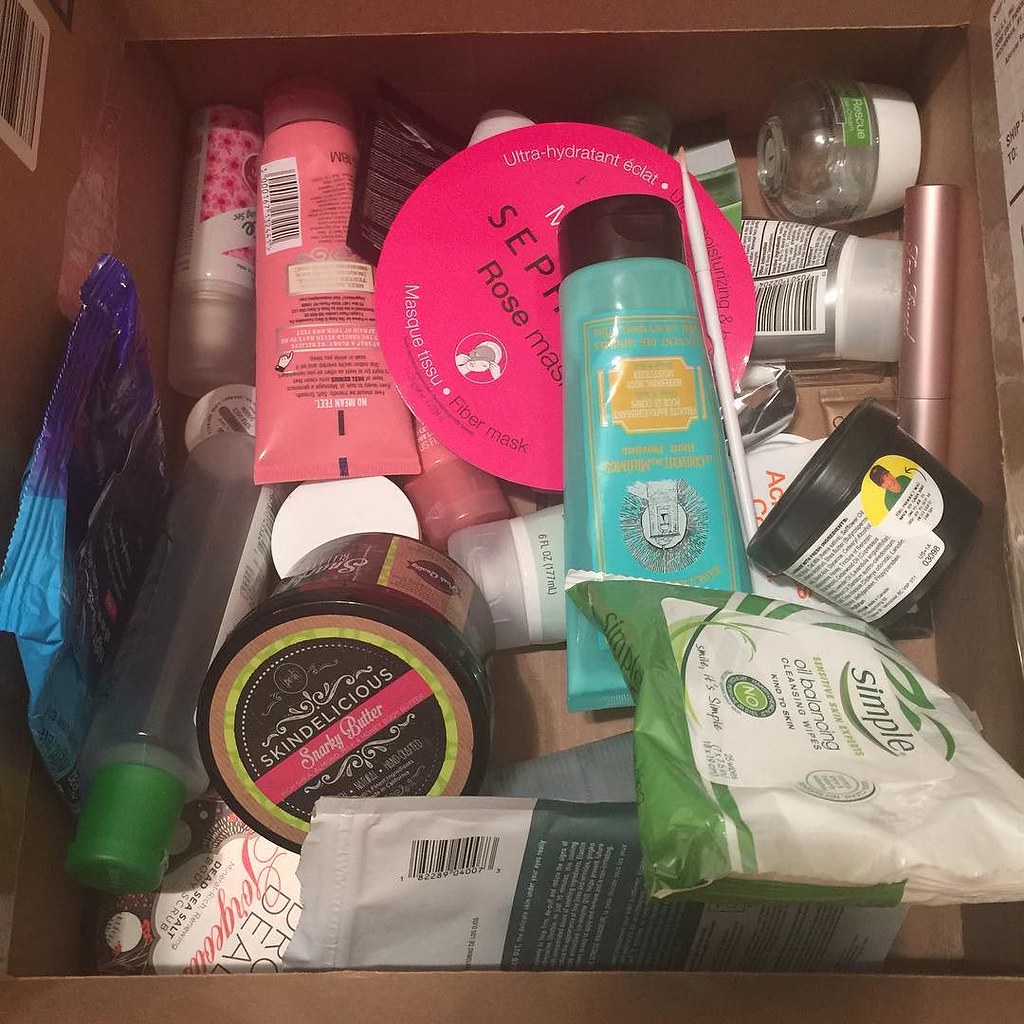In the image, there is an array of various containers organized within a larger container that has visible brown walls at the bottom. Starting at the top, a blue squeeze tube with yellow lettering is noticeable, though the text is not readable. Below this is a pink circular package labeled "Sephora Rose Mask". To its left, the back of a pink squeeze tube with black lettering and a black and white barcode is partially visible. Nearby, a small can of Batiste hairspray in pink floral packaging can be identified even though the brand name isn't visible. 

At the bottom right, there is a white and green plastic package of Simple Sensitive Skin Experts Oil Balancing Cleansing Wipes, labeled "kind to skin". Above these wipes, a black plastic container with a screw-off top, likely a Lush product, has a white label with black lettering and a circular label featuring a person's face on top.

Above this, there is a pink tube of mascara, possibly from the Too Faced brand. On the bottom left, a black tub labeled "Skin Deletion Snarky Butter" suggests it contains body butter. Beside it, an almost empty clear plastic bottle with a green top, presumably for makeup remover, stands next to an overturned blue plastic package with illegible text.